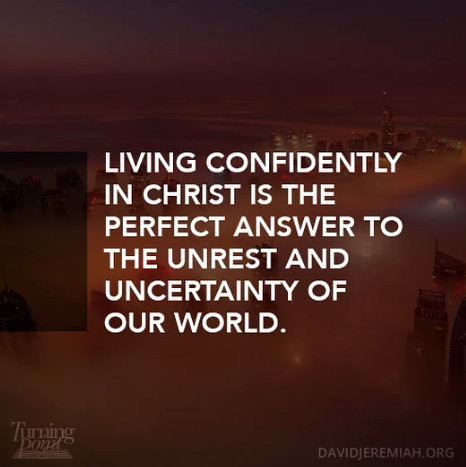This religious advertisement features a predominantly dark reddish-brown sky with a faint, shadowy image of religious structures or a cityscape in the background, shrouded in fog or mist. The poster's emphasis is on an inspirational quote, boldly displayed in white lettering at the center: "Living confidently in Christ is the perfect answer to the unrest and uncertainty of our world." The lower left corner of the poster reads "Turning Point," while the lower right corner displays "DavidJeremiah.org." The design aims to provide hope and encouragement amidst the depicted ominous, cloudy atmosphere.